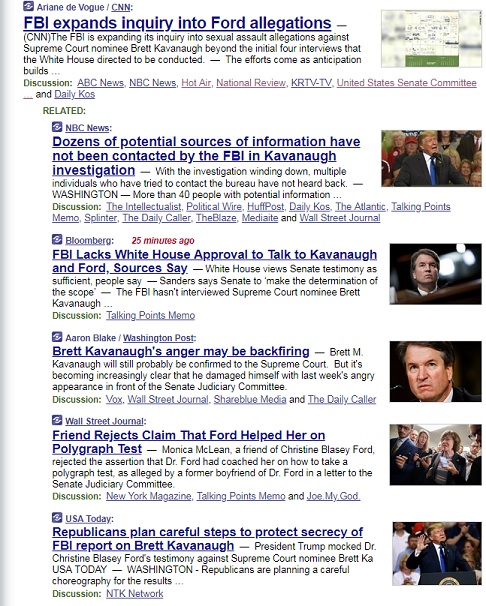**Detailed Descriptive Caption:**

A search results webpage for news information is displayed. At the top of the results, an article by **Ariane de Vogue from CNN** is highlighted with the headline: **"FBI expands the inquiry into foreign allegations."** Directly below, additional search results are listed with headlines from various news sources. Detailed tabs at the top of the page allow switching to different new outlets: **ABC News, NBC News, Hot Air (highlighted in red), National Review (highlighted in red), KRTV-TV, United States Senate Committee (highlighted in red), and Daily Calls**. 

Related articles are listed with the following headlines and sources:
1. **NBC News** - "Dozens of potential sources of information have been contacted by the FBI in the Kavanaugh investigation."
2. **Bloomberg - 25 Minutes Ago** - "FBI lacks White House approval to talk to Kavanaugh and Ford says source."
3. **Washington Post** - "Brett Kavanaugh's anger may be backfiring."
4. **Wall Street Journal** - "Friend rejects claim that Ford helped her on polygraph test."
5. **USA Today** - "Republicans plan careful steps to protect the secrecy of FBI report on Brett Kavanaugh."

An image accompanying the search results shows former President Trump at a podium, adding a curious visual element to the page. The highlighted tabs (Hot Air, National Review, and United States Senate Committee) suggest these are currently selected or popular sources.